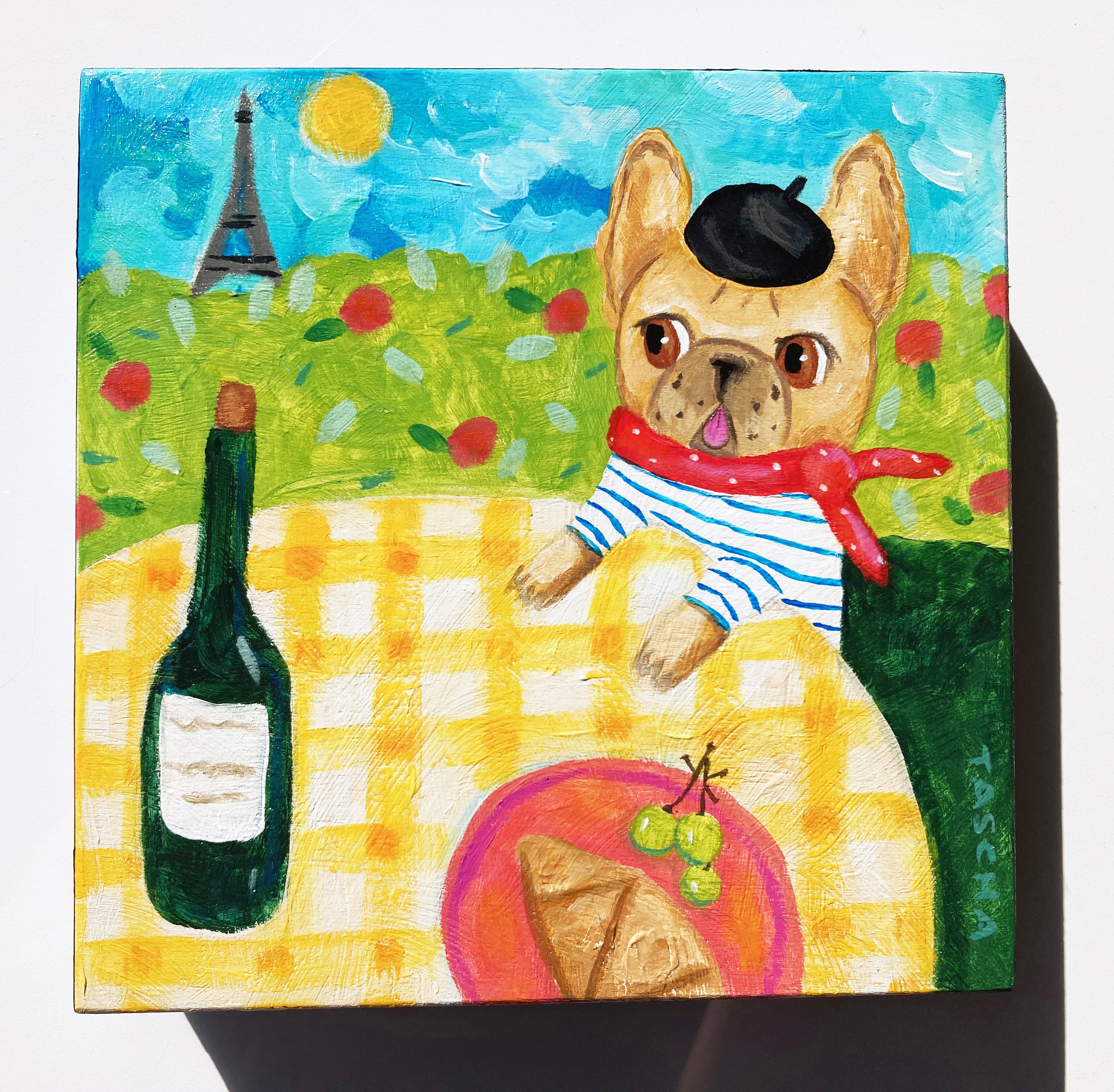This charming painting, created by Tasha Parkinson, portrays a delightful Parisian scene featuring a small light brown French bulldog adorned in quintessential French attire. The dog wears a black beret, a blue and white striped shirt, and a red handkerchief around its neck, while seated at a yellow and white gingham-covered table. Before the dog, on the table, rests a red plate holding a croissant and three green grapes, beside a dark green wine bottle. The dog gazes to its right with its tongue playfully out, ready for a snack. Behind the dog, there is a lush green bush dotted with bright pink flowers and red fruits, set against a backdrop of a light blue sky with clouds. In the distance, the iconic Eiffel Tower stands tall with the sun shining to its right. The artwork, featuring a childlike, amateurish style, is signed "Tasha" vertically on the bottom right.